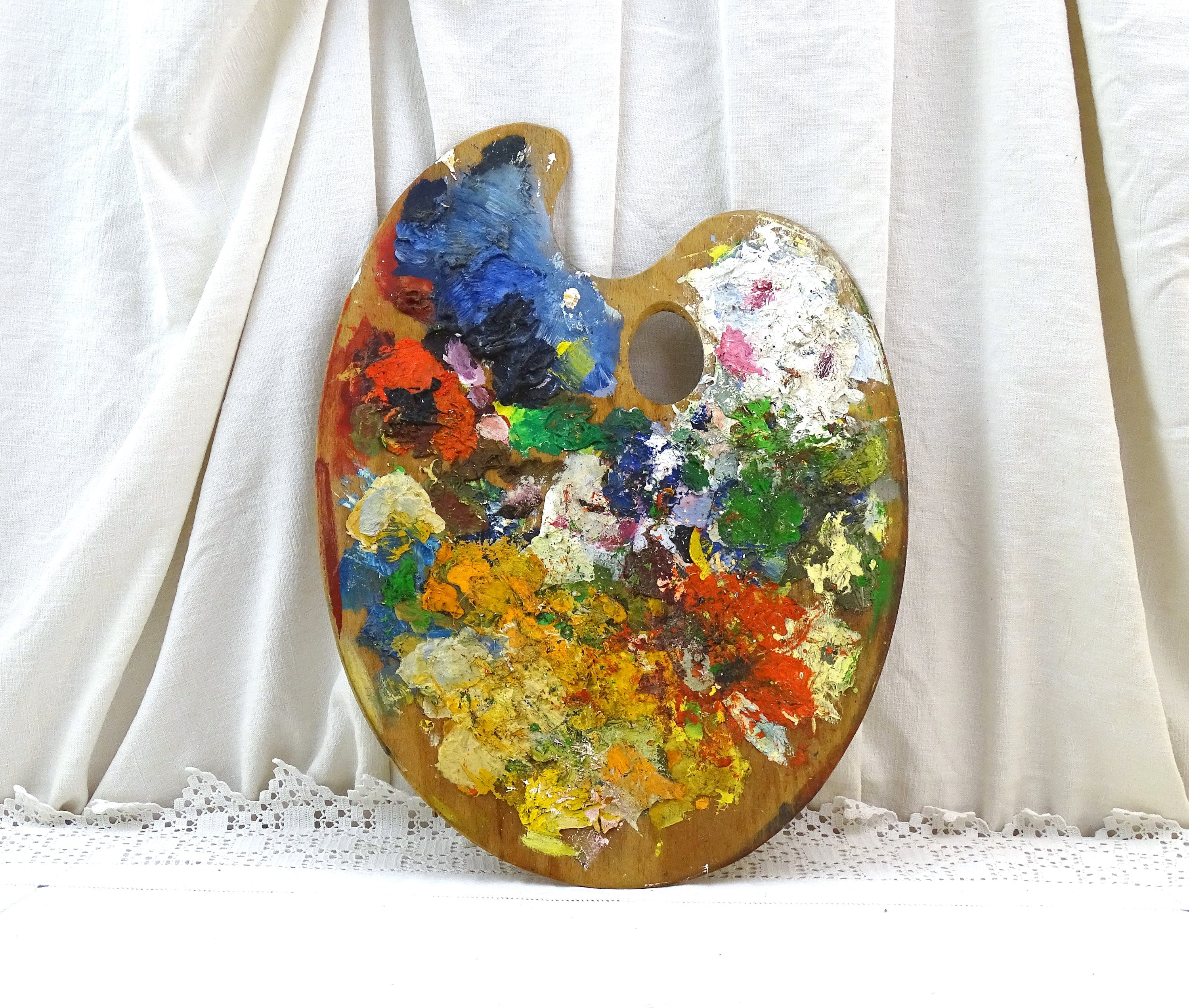This image captures a well-used artist's palette, a familiar wooden board with a distinctive thumb hole, allowing the painter to hold it with ease. The palette is prominently coated with a wide spectrum of vibrant colors, including blue prominently in the upper portion, a blend of white and pink in the top right, and various shades of yellow, orange, and green. Notably, there's a lot of red distributed throughout the palette. The circular design features another cutout for resting the forearm. This well-worn palette leans against a dolly or a table draped in white fabric, situated on the floor against a wall adorned with white curtains, adding a soft backdrop to the scene.